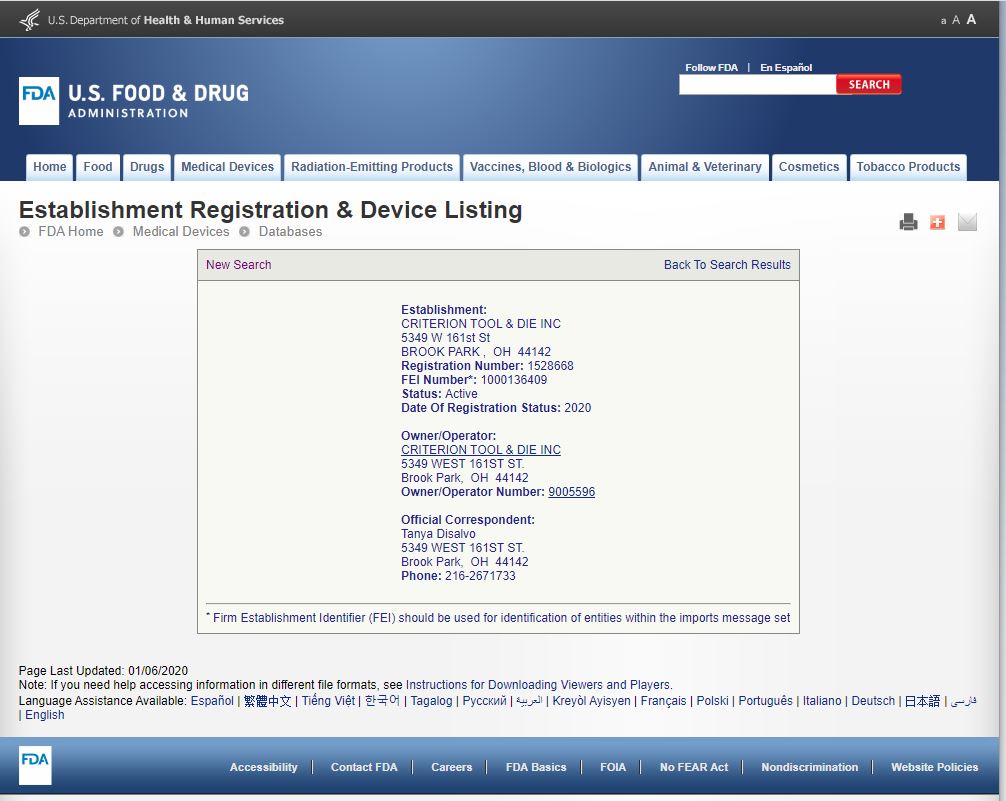This is a webpage from the U.S. Food and Drug Administration (FDA). The title bar in the upper left reads "U.S. Department of Health and Human Services," and directly below, the main header of the website displays the FDA logo alongside the text "FDA, U.S. Food and Drug Administration." To the right of this title, a search box is present, accompanied by a red search button. Above the search box, there are links for following the FDA on various platforms and a button labeled "En Español" for switching the website language to Spanish.

The main body of the webpage indicates the section for "Establishment Registration and Device Listings." Breadcrumb navigation shows links to "FDA," "Home," "Medical Devices," and "Databases." A search result box is displayed, revealing that a search has been conducted for "Establishment Criterion Tool and DIEG." 

The search result provides the address "349 West 61st Street, Brook Park, Ohio, 44142," along with the registration number, FEI number, status, and date of the registration status. The entry identifies Criterion Tool and DIEG, Inc. as the owner-operator. This specific registration and device listing pertains to Criterion Tool and DIEG, Inc.